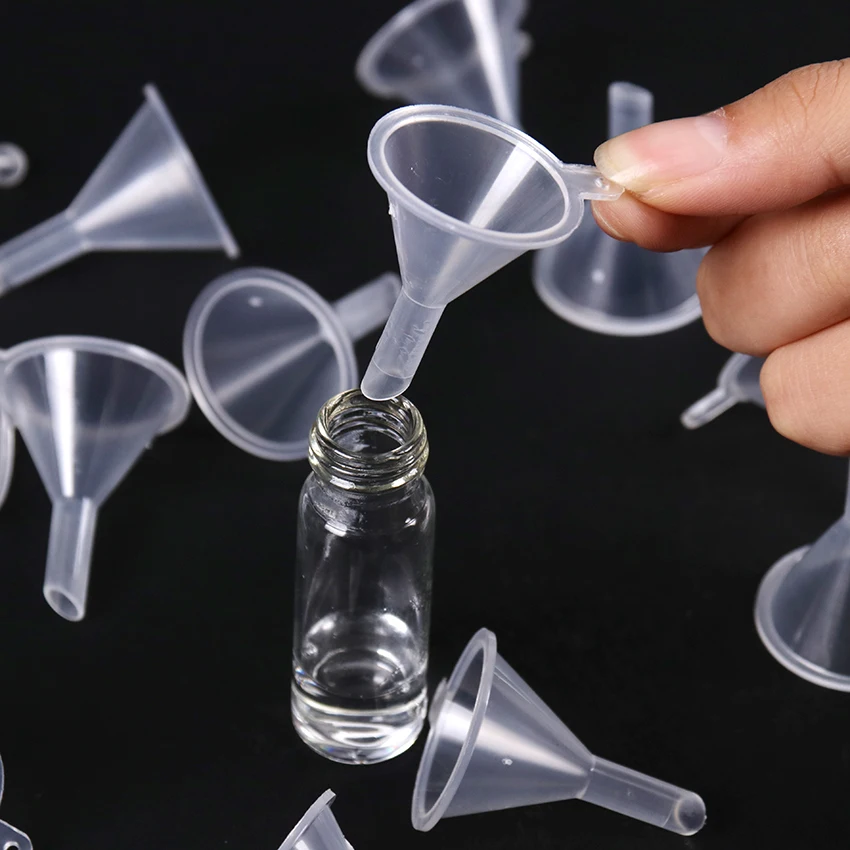The photograph, styled like a catalog or advertisement, features a pitch-black background, contrasting sharply with the central subjects. In the center of the image is a small, narrow glass bottle containing a clear liquid. Above the bottle's mouth, a white female hand with slightly longer nails delicately holds a tiny, clear plastic funnel using the thumb and index finger by its handle. The focus is on this hand-funnel-bottle combination, emphasizing the small size and precision of the items. Surrounding the central setup, numerous similar clear plastic funnels are scattered in various positions on the black background, some lying on their sides, others upside down, adding to the composition's sense of casual disarray. The funnels appear to be haphazardly dropped, further highlighting the in-focus funnel being held above the bottle.